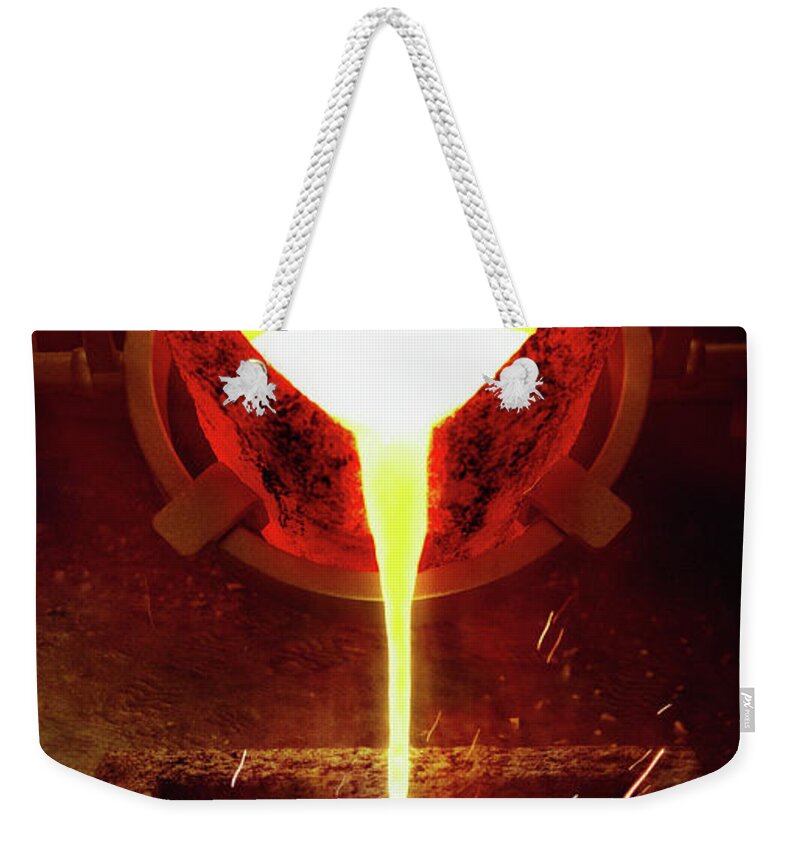The image features a striking handbag, likely a tote bag, with a vivid screen-printed design that depicts a molten metal pouring scene. The bag's handle is crafted from a white braided cord, which threads through two grommets at the top, forming a secure, somewhat fluffy knot at each end where it emerges inside the bag. The dynamic graphic portrays molten liquid, perhaps steel or metal, cascading from a container, suggesting a fiery furnace or a smelting process. The liquid appears to be pouring onto or near a wooden log, with accompanying sparks flying up, enhancing the dramatic effect. The lower part of this vivid illustration features what looks like a metallic bowl or vessel containing molten metal. Additionally, there's a small, unreadable tag on the side of the bag, possibly indicating the brand. The overall design may symbolize the duality of the creation process and the finished product, blending industrial elements with artistry.